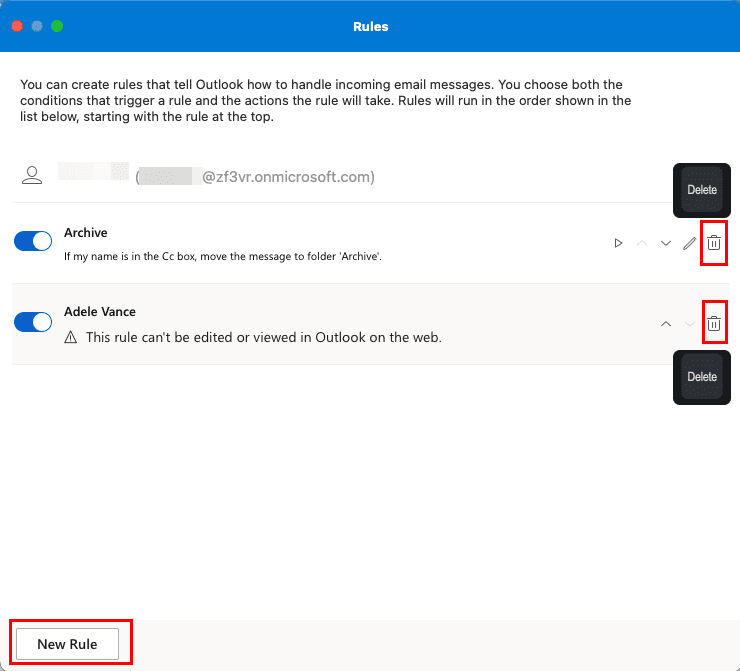This image is a detailed screenshot from a tutorial on setting up or configuring the Outlook email client. 

At the top, a prominent blue banner stretches across the screen. Within this banner, three dots on the left—colored red, blue, and green—are displayed, while the centered white text reads "Rules."

Below the banner, the screen transitions to a white background with black text. The first paragraph explains the functionality: "You can create rules that tell Outlook how to handle incoming email messages. You choose both the conditions that trigger a rule and the actions the rule will take. Rules will run in order shown in the list below, starting with the rule at the top."

A small blank profile icon of a person and a concealed email address (zf3vr.onmicrosoft.com) appear toward the top left beneath this text. To the right of this profile information, there is a prominent black button labeled "Delete."

Displayed further down is a section for configuring rules. One such rule labeled "Archive" is currently selected. The corresponding description for this rule reads: "If my name is in the CC box, move the message to folder Archive." Adjacent to this rule are several icons including a play button, an up and down arrow, a pencil for editing, and a trash can. The trash can icon is highlighted with a red box.

Following the "Archive" rule is another rule labeled "Adele Vance." This rule is also selected and flagged with a triangular warning sign. The description notes: "This rule can't be edited or viewed in Outlook on the web." Similar to the previous rule, the same set of icons is present, with the trash can icon again circled in red.

At the bottom left corner of the screen is a noticeable white button labeled "New Rule," which is also circled in red, indicating its importance in the tutorial.

This comprehensive screenshot serves as a clear visual aid for users learning to create and manage rules in Outlook.